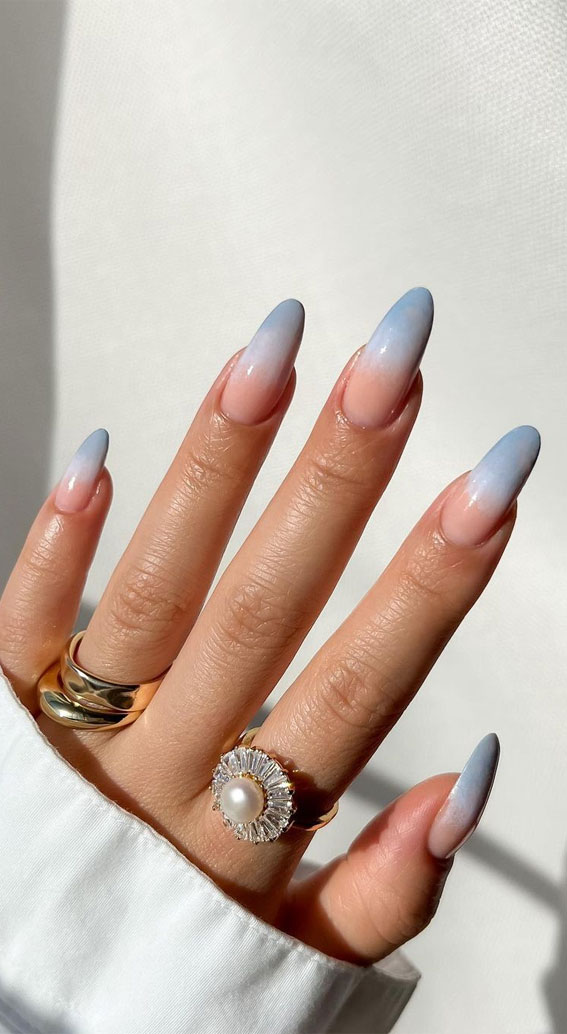In the image, the focus is on an elegantly manicured hand with long, pointy fingernails adorned with a unique gradient of colors—bluish tips, a whitish middle section, and reddish areas near the cuticles. The hand features two distinctive rings: one on the ring finger is an intricate design with interlocking silver and gold loops, while the index finger sports a floral ring with detailed petal engravings centered around a small pearl, set in a gold band. The hand is partially covered by a white sleeve that reaches close to the fingers, adding a touch of sophistication. The background is a simple white, with a subtle shadow creating depth and focusing attention on the hand.